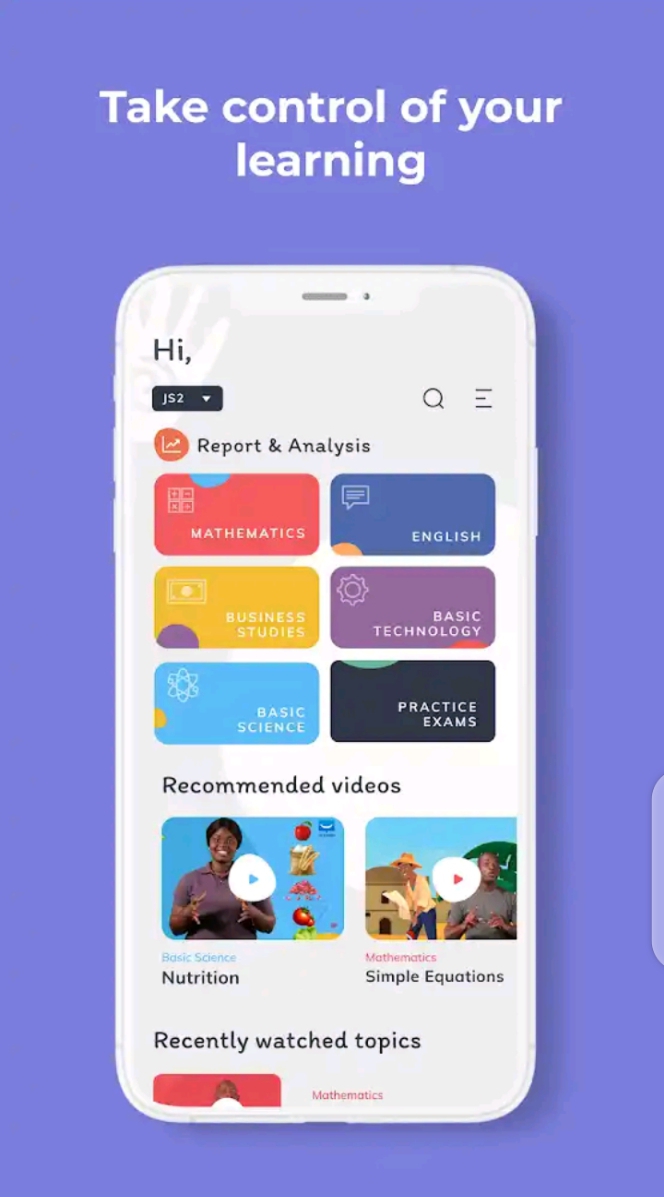The image features a prominently titled purple box at the top, with the text "Take Control of Your Learning" displayed in white. Below this header, a smartphone icon is positioned against a gray background adorned with white handprints. The smartphone screen shows various elements including a greeting that says "Hi," a black drop-down menu, a magnifying glass icon, and a red circular button labeled "Report and Analysis."

Beneath these elements, subject-specific buttons are arranged in a grid layout. From left to right and top to bottom, the buttons are as follows:
- A red rectangle labeled "Mathematics."
- A blue rectangle labeled "English."
- A yellow rectangle labeled "Business Studies."
- A purple rectangle labeled "Basic Technology."
- A light blue rectangle labeled "Basic Science."
- A black rectangle labeled "Practice Exams."

Further down, the section titled "Recommended Videos" showcases two video thumbnails, each with a play icon in the center. The first thumbnail on the left is captioned "Nutrition," while the second thumbnail on the right is titled "Simple Equations." Below this, the section is labeled "Recently Watched Topics."